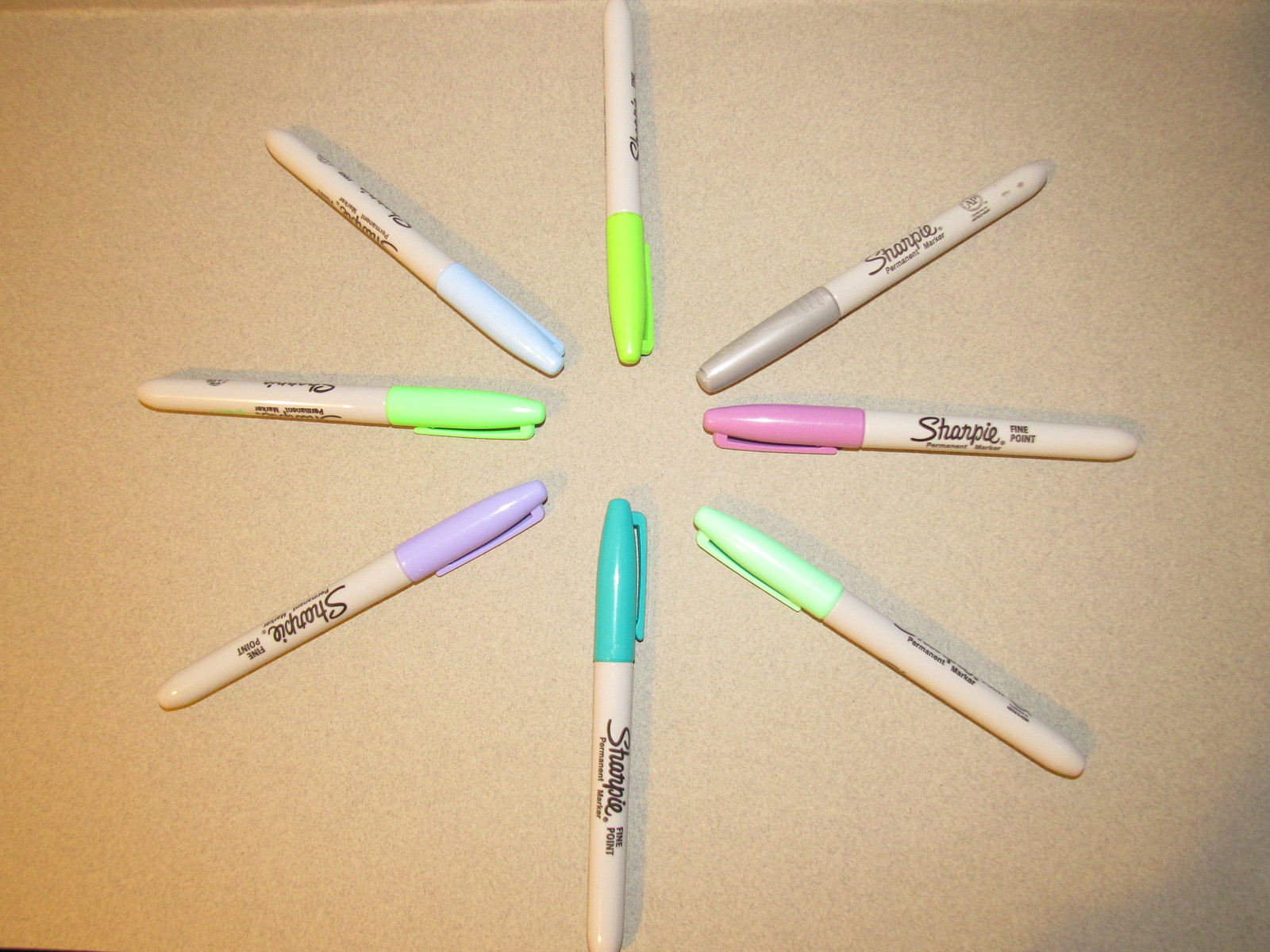The photograph depicts eight Sharpie markers arranged in a star formation on a light, possibly cream-colored surface. All the Sharpies have light gray bodies with the "Sharpie" branding prominently displayed in black. The caps of the markers, which are pointed inward, are varied and vibrant in color. Starting from the marker at the top and moving clockwise, the caps are neon lime green, silver, bright pink, seafoam green, teal, lavender purple, mint green, and pastel periwinkle blue. Each cap's unique color suggests that the Sharpies themselves are likely of the corresponding colors. The arrangement and distinct color caps create an eye-catching, symmetrical pattern, making the workspace both colorful and organized.